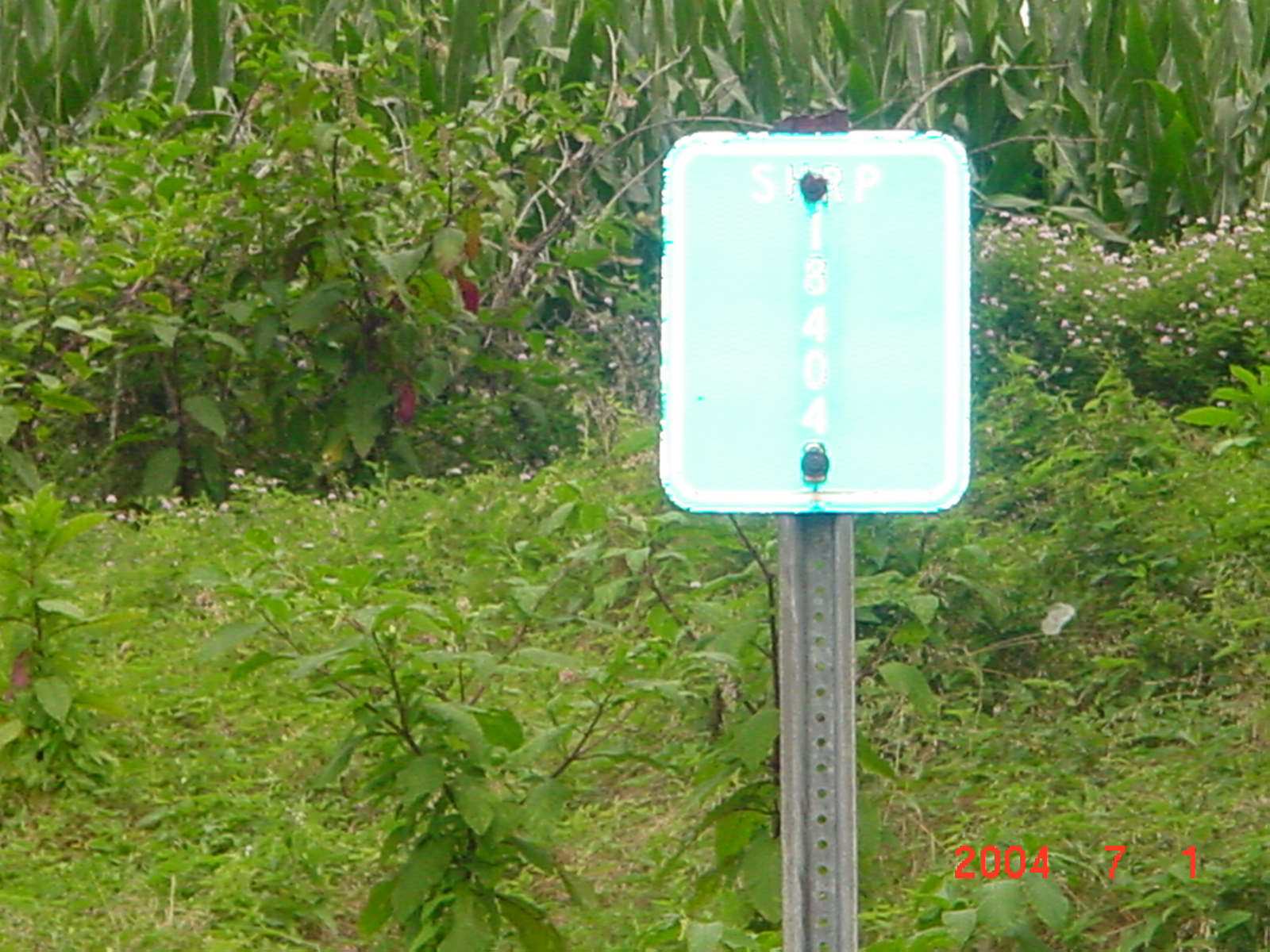This color photograph captures a close-up view of a highway sign set amidst a lush, green environment. The sign, mounted slightly off-center to the right on a vertical steel bar with perforations, is prominently featured. It is an old, faded green with a white border and slightly curved edges, and it appears reflective. The text on the sign includes "S&P" at the top, partially obscured by a rivet, and the number "18404" running vertically down the center. Another date, "7-1-2004," is visible to the right. The backdrop is densely packed with various types of greenery, including tall grasses, bushes, and numerous leaves and branches. Among the plants, there are some white flowers, tiny pink flowers, and purple blooms interspersed, contributing to the verdant and somewhat overgrown scene. The overall setting suggests an area rich with vegetation, where the sign stands as the central focus amidst the natural surroundings.